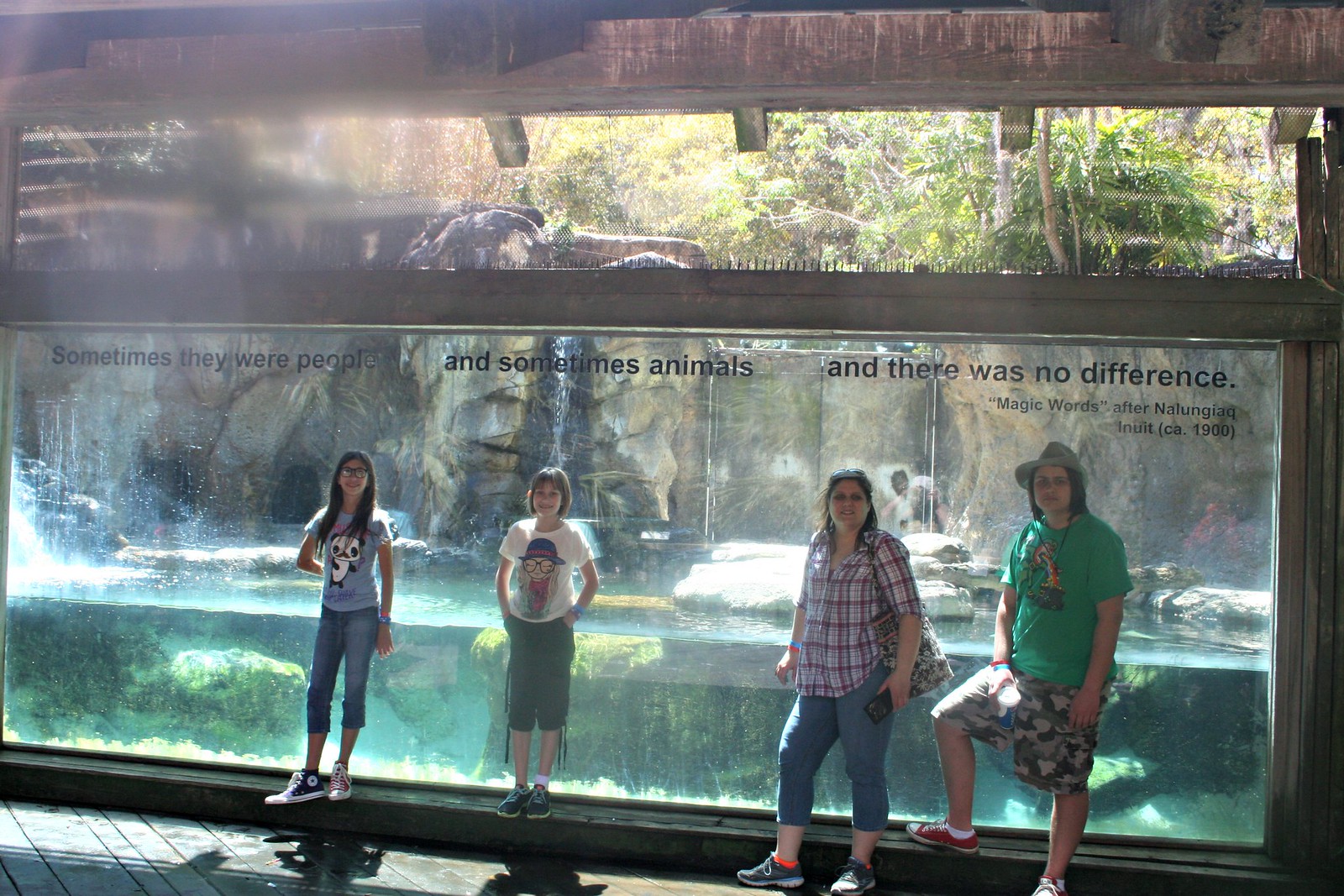This daytime photograph, taken inside an aquarium or zoo exhibit, captures a family of four standing in front of a large glass window. The exhibit behind the glass appears to be a meticulously crafted natural habitat featuring water, rock formations, and trees. No animals are visible, but it might house aquatic life such as alligators or amphibians. The glass window bears an inscription: "Sometimes they were people and sometimes animals, and there was no difference. Magic words after Nutagwan Inuit, circa 1900."

The sunlight illuminates the scene, casting a warm glow. The four individuals include two young girls, an older woman, and an older man, each wearing wristbands indicative of their entry into the location. The girl on the left sports a blue top with a cartoon character, blue jeans, mismatched sneakers in black and red, glasses, a wristband, and a wristband. The other girl has short blonde hair, a white top with a girl's image, green quarter pants, and sneakers. The older woman, equipped with a jacket, blue jeans, sport shoes, a bag, smartphone, and sunglasses atop her head, is also wearing the wristband. The older man, possibly not the father, is dressed in a green t-shirt, a hat, camouflage shorts, red canvas shoes, and is holding a cold drink cup, while also wearing the wristband. The family appears to be enjoying their visit and posed specifically for this photograph. The overall image has a slightly blurry quality but captures a vivid moment of family bonding and curiosity.